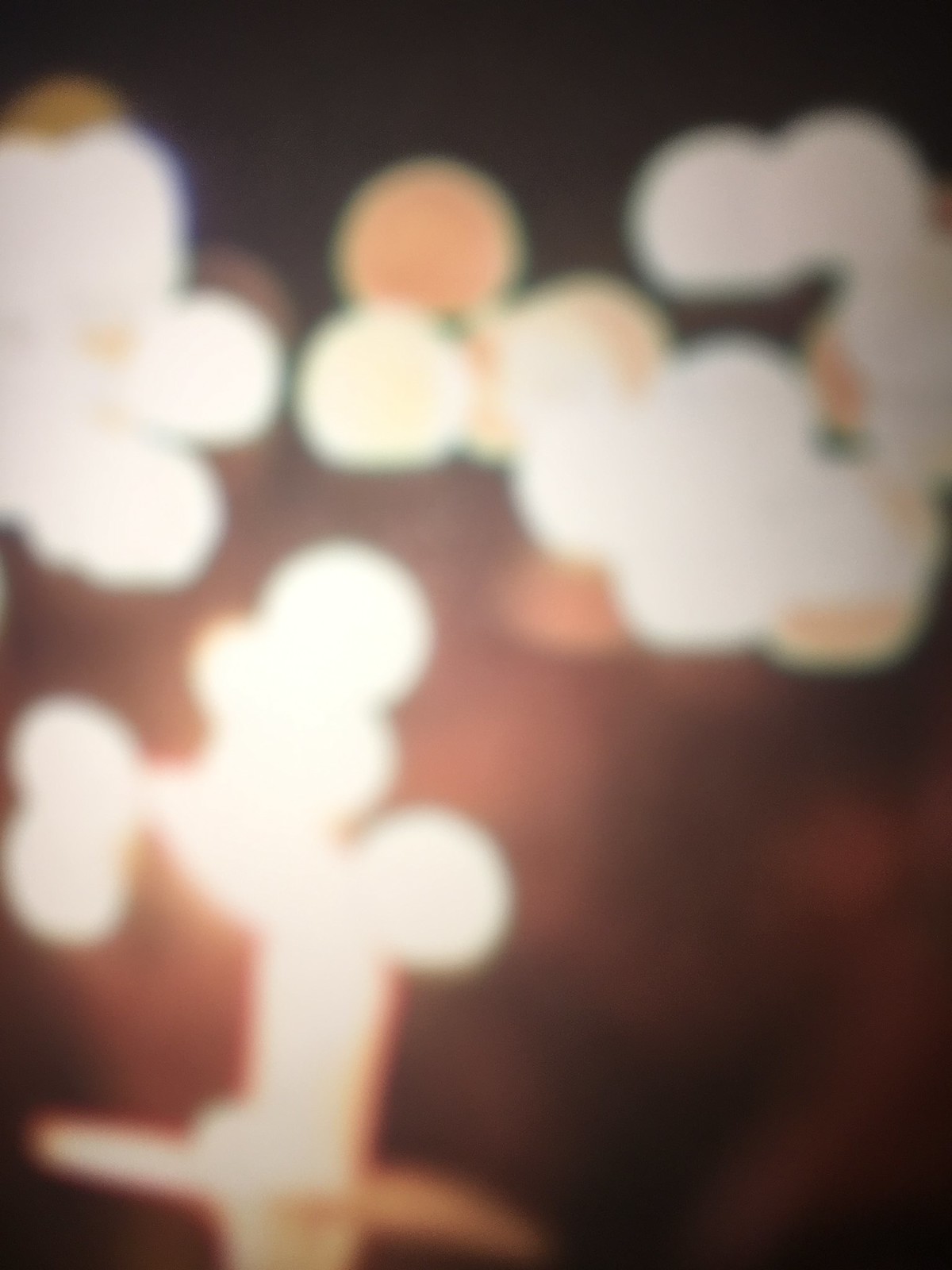A nighttime photograph featuring a softly blurred array of lights against a dark backdrop. The bright lights, varying in intensity, include several small, glowing orbs that give off a distinct orange hue. The overall effect is a dreamy, abstract representation of a night scene, where the identity of specific objects remains indistinguishable.